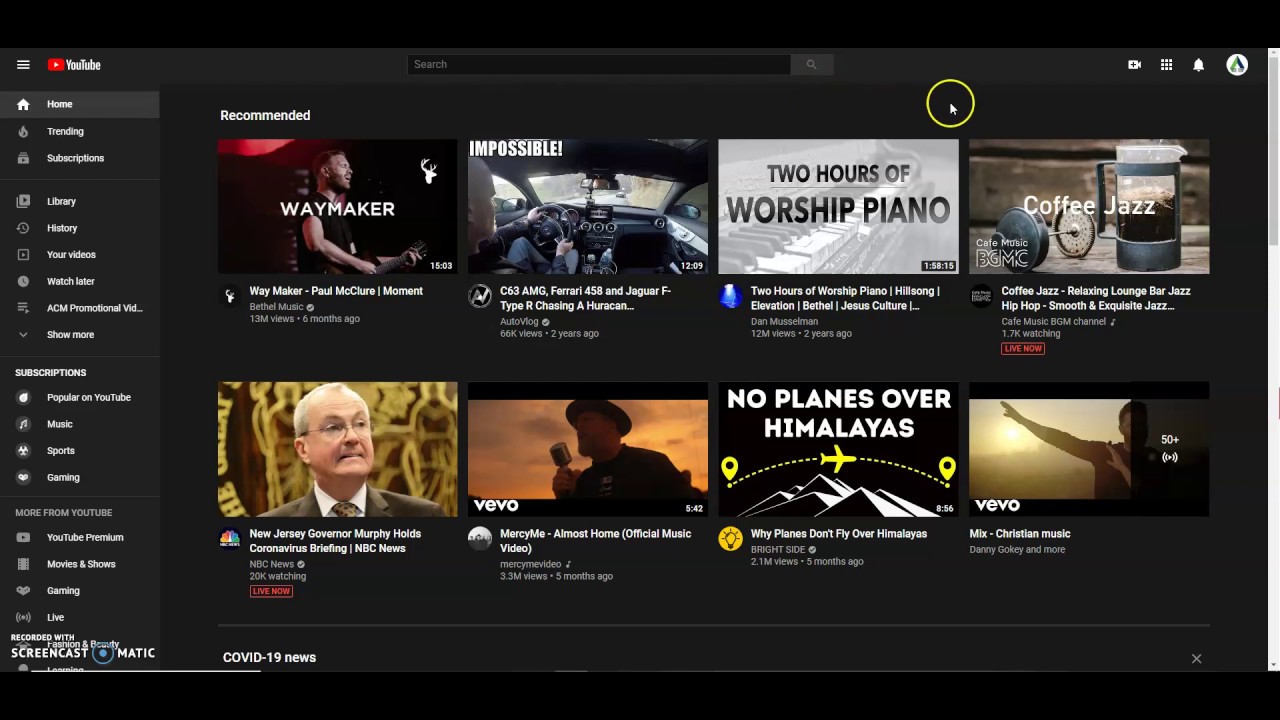The image showcases a computer screen displaying the YouTube homepage. The interface has a sleek black background. In the upper left corner, three horizontal white lines signify the main menu. Adjacent to this, the YouTube logo is prominently displayed, with the word "YouTube" in white set against a red play button symbol. 

Below the logo are various menu options with corresponding icons:
- **Home**: Represented by a house icon.
- **Trending**: Symbolized by a fire icon.
- **Subscriptions**: Marked with an arrow button.
- **Library**: Indicated by an advance button.
- **History**: Shown with a circular arrow icon.
- **Your Videos**: Depicted as a square icon.
- **Watch Later**: Denoted by a clock icon.

Further down the screen, a section titled "ACM promotional vid" is visible, followed by a pointer icon suggesting to "Show more." Under the "Subscriptions" header, written in bold white letters, are various categories like "Popular on YouTube," "Music," "Sports," and "Gaming." The "More from YouTube" heading, colored in gray, lists additional options including "YouTube Premium," "Movies and shows," "Gaming," and "Live," each accompanied by small icons.

The main content area features eight video thumbnails:
1. **Waymaker**: A thumbnail showcasing a singer.
2. **C63 Ferrari 458 and Jaguar F Type R chasing a hurricane**: An image of someone inside a car.
3. **Two Hours of Worship Piano**: A piano keyboard set against a gray background with the title in black.
4. **Coffee Jazz**: Displays a French press with its top pulled out.
5. **New Jersey Governor Murphy holds coronavirus briefing, NBC News**: An older man with gray hair.
6. **Vivo, Mercy Me - Almost Home**: A man holding a microphone against a golden sky.
7. **No planes over Himalayas**: A graphic of mountains with a small yellow plane and dotted lines.
8. **Vivo - Mix of Christian Music**: A scene featuring the sun in the background and a man's raised arms.

Overall, the screen captures a richly detailed and organized snapshot of the YouTube platform.